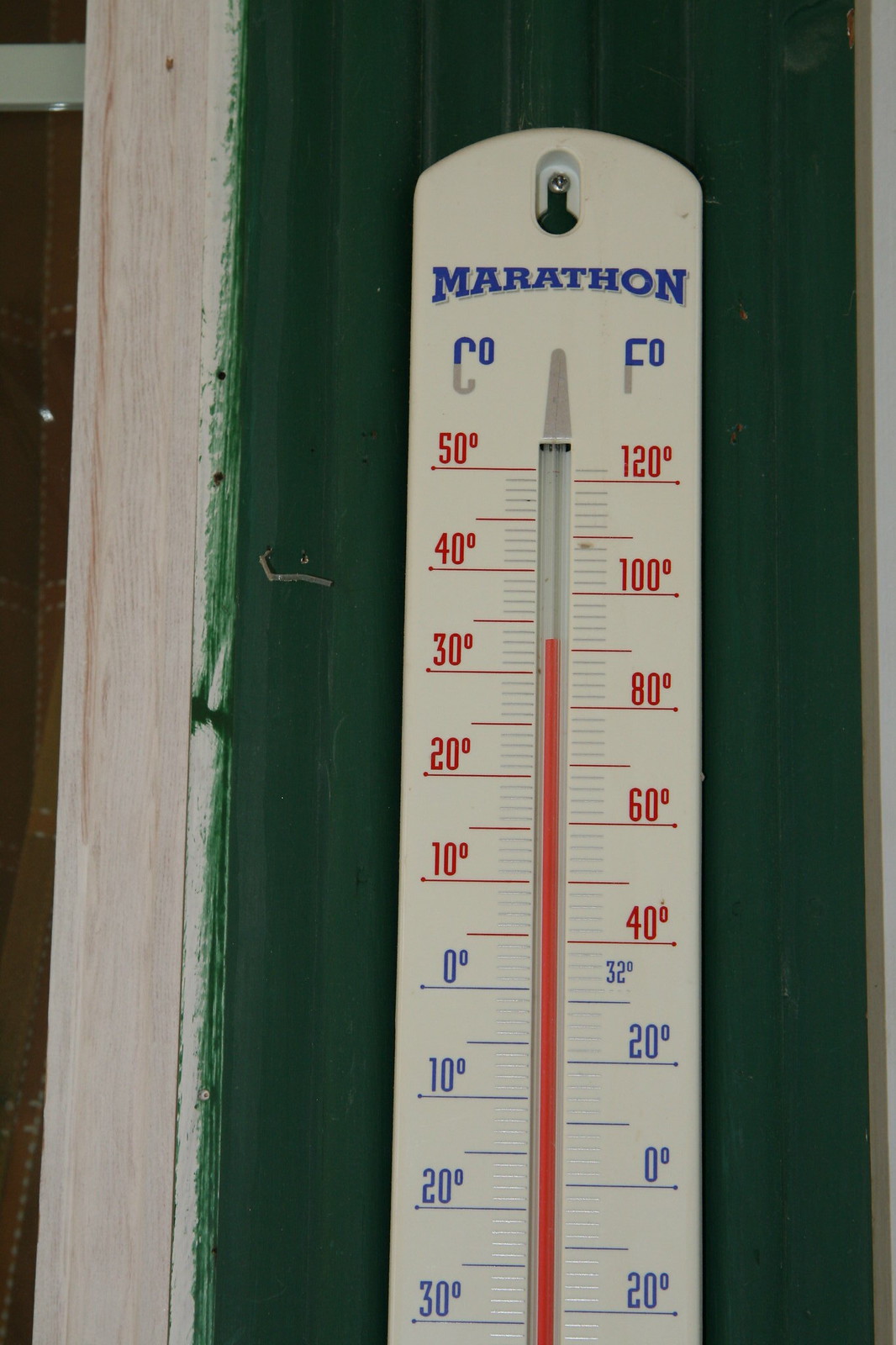A white, rectangular-shaped thermometer with a curved top is mounted on a green wall that appears to be poorly painted; some green paint has overlapped onto a white section. The thermometer displays the brand name "Marathon" in blue. The current temperature is approximately 85 degrees Fahrenheit (30-32 degrees Celsius). The temperature readings are in red above 32°F and turn blue below that mark. On the left side of the image, part of a brown wall is visible. The green wall has a noticeable small scratch running through it, adding to the imperfect aesthetic of the setting.